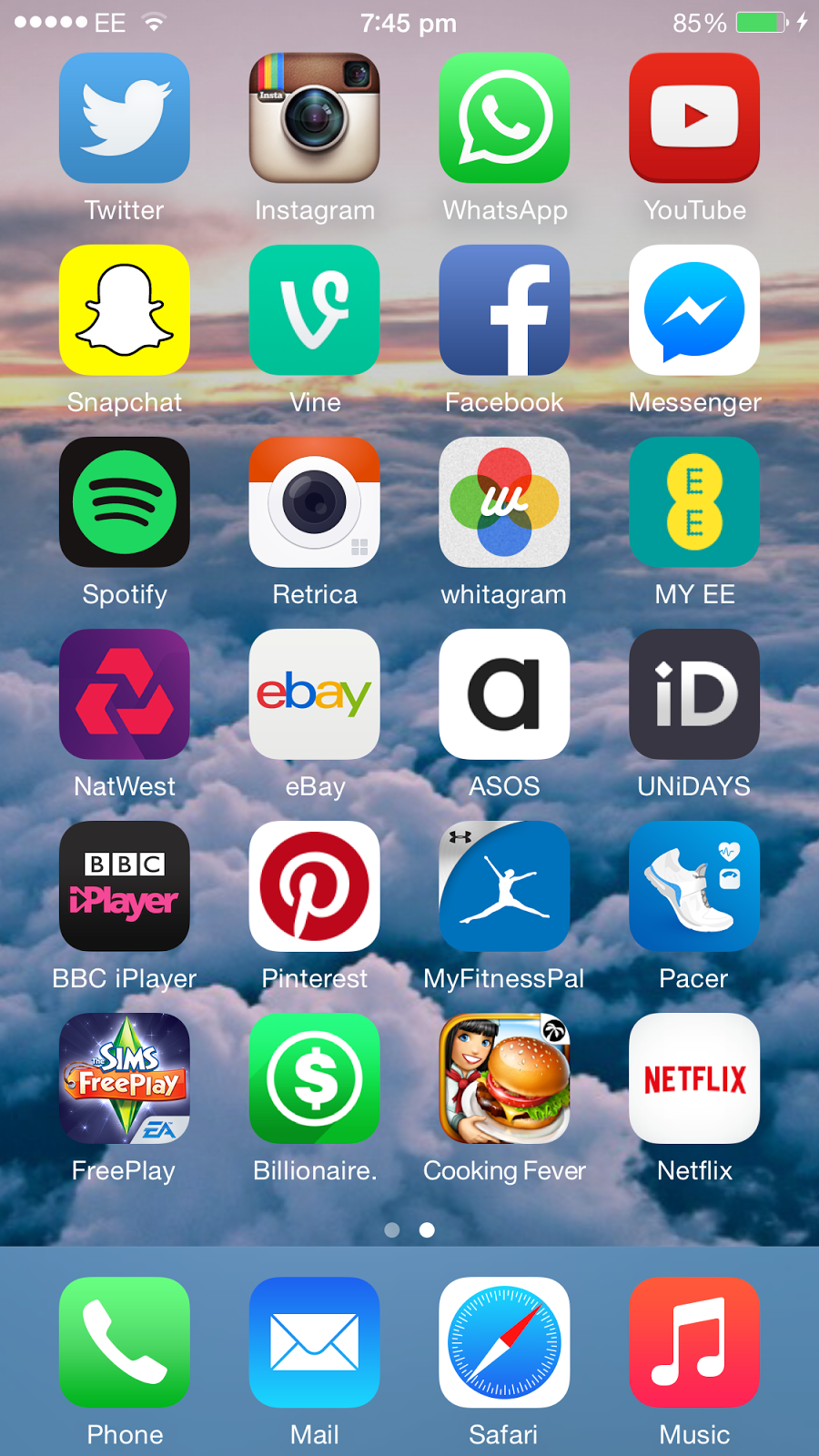The image showcases a smartphone home screen with various app icons. At the top of the screen, the time displayed is 7:45 PM, with a battery icon showing 85% charge and actively charging. A Wi-Fi icon is also visible. 

The home screen is populated with several app icons, each distinct in color and design:

- **Twitter**: Blue and white icon
- **Snapchat**: Yellow and white icon
- **Spotify**: Black and green icon
- **NatWest**: Purple and red icon
- **BBC iPlayer**: White, pink, and red icon
- **The Sims FreePlay Billionaire**: White and green icon
- **Pinterest**: Red and white icon
- **Google Maps (likely referring to IPA)**: Red, blue, yellow, green, and white icon
- **Red Reading**: White and orange icon (possibility of misidentification)
- **Instagram**: Icon featuring a camera image
- **Facebook**: Blue and white icon
- **Google Search (referred to as 'white cream')**: Red, green, blue, and yellow icon
- **Sauce (possibly an error, may refer to an app like 'Slack')**: White and black icon
- **MyFitnessPal**: Blue and white icon with grey
- **Cooking Fever**: Icon with a picture of a burger
- **Netflix**: Red and white icon
- **PayPal/Samsung Pay (referred to as 'PESA')**: Blue icon
- **Unidays**: Black and white icon
- **My EE**: Green and yellow icon
- **Messenger**: White and blue icon
- **YouTube**: Red and white icon

At the bottom of the screen, there are additional icons:

- **Phone**: Green and white icon located at the bottom left corner
- **Mail**: Blue and white icon
- **Safari web browser**: White and blue icon featuring a needle (compass)
- **Music**: Red and white icon

The smartphone home screen is a vibrant array of applications that provide a wide range of functionalities, from social media and entertainment to utility and fitness tracking.